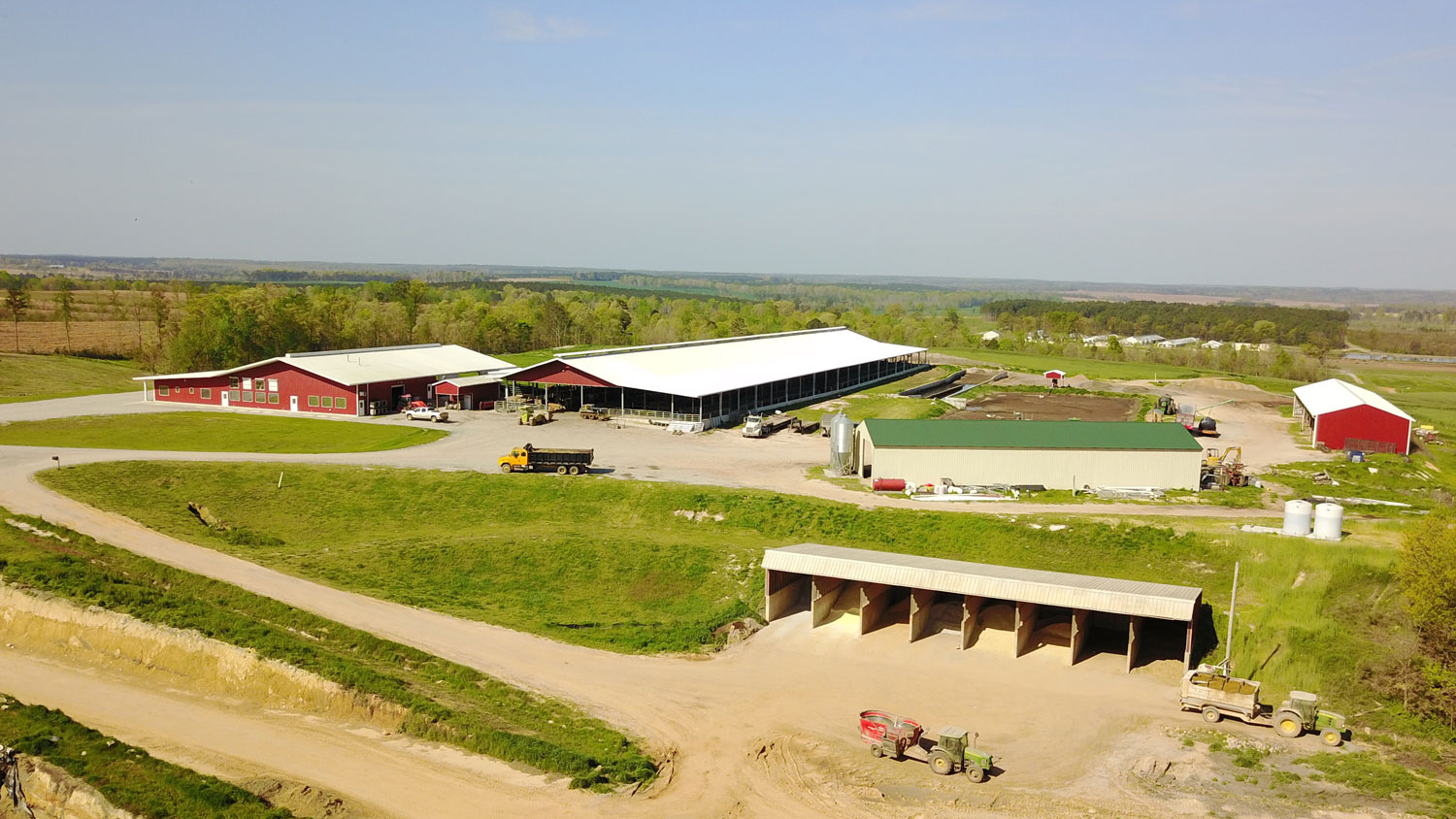The photograph presents an aerial view of a sprawling farm set in a flat landscape under a grayish-blue sky. Dominating the scene are four barns: two on the left with red siding and white roofs, and two on the right, one with white siding and a green roof, and the other with red siding and a white roof. The long barns feature triangular rooftops and extend far into the distance. The one with open walls appears suited for animal housing, while another one has closed walls. Numerous gravel and dirt roadways meander through the property, with a few trucks and tractors visible—one, a yellow truck with a black bed, and another, a green tractor pulling a red object. Further details include a gray garage area with multiple ports and another green tractor with yellow wheels towing something gray. In the foreground, there are empty animal pens, while trees and expanses of brown field mark the background, providing a serene horizon.